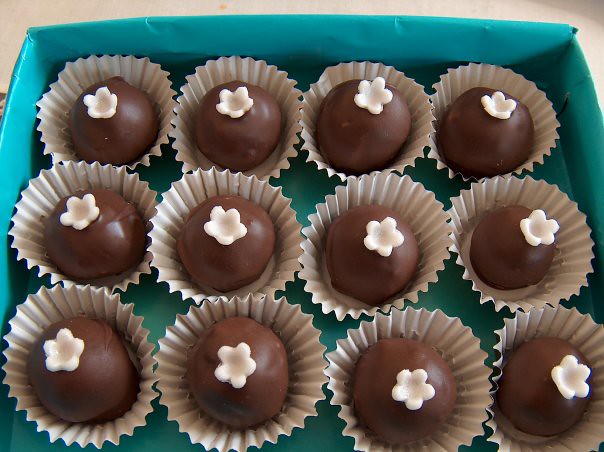This indoor color photograph captures a neatly arranged set of twelve chocolate treats inside an open teal box. Each round, half-spherical chocolate candy rests in a white cupcake holder, showcasing a delicate white, five-petal flower ornament on top. The candies, presented in three rows of four, have a smooth, untouched surface, indicating their pristine condition. The teal box, though utilitarian in appearance, serves to conveniently store and transport the chocolates. The backdrop visible in the upper corners of the photograph is a plain white, ensuring all focus remains on the intricately detailed candies within the well-lit image.